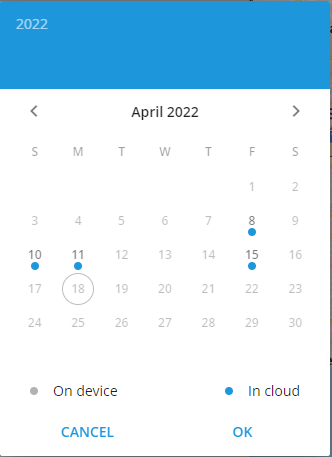The image depicts a digital screen displaying a calendar interface with a blue banner along the top. In the upper left corner of the banner, the year "2022" is prominently featured in white text. The main section of the screen presents the calendar for April 2022, with navigation arrows on either side allowing users to switch to the previous or subsequent months.

The calendar is formatted in a traditional layout, beginning with Sunday on the far left and ending with Saturday on the far right. The dates are indicated by numbers below each day of the week. Notably, several dates are highlighted with specific markers: the 8th, 10th, 11th, and 15th have small blue dots below their numbers and are slightly bolded. The 18th is distinctly marked with a circle around the date.

At the bottom of the calendar, a legend clarifies the meaning of these symbols: a blue dot indicates that the event is stored in the cloud, while a circle signifies that the event is saved on the device. Beneath this legend, two blue buttons are positioned side-by-side, with a "Cancel" button on the left and an "OK" button on the right, providing the user with options to either dismiss or confirm their actions.